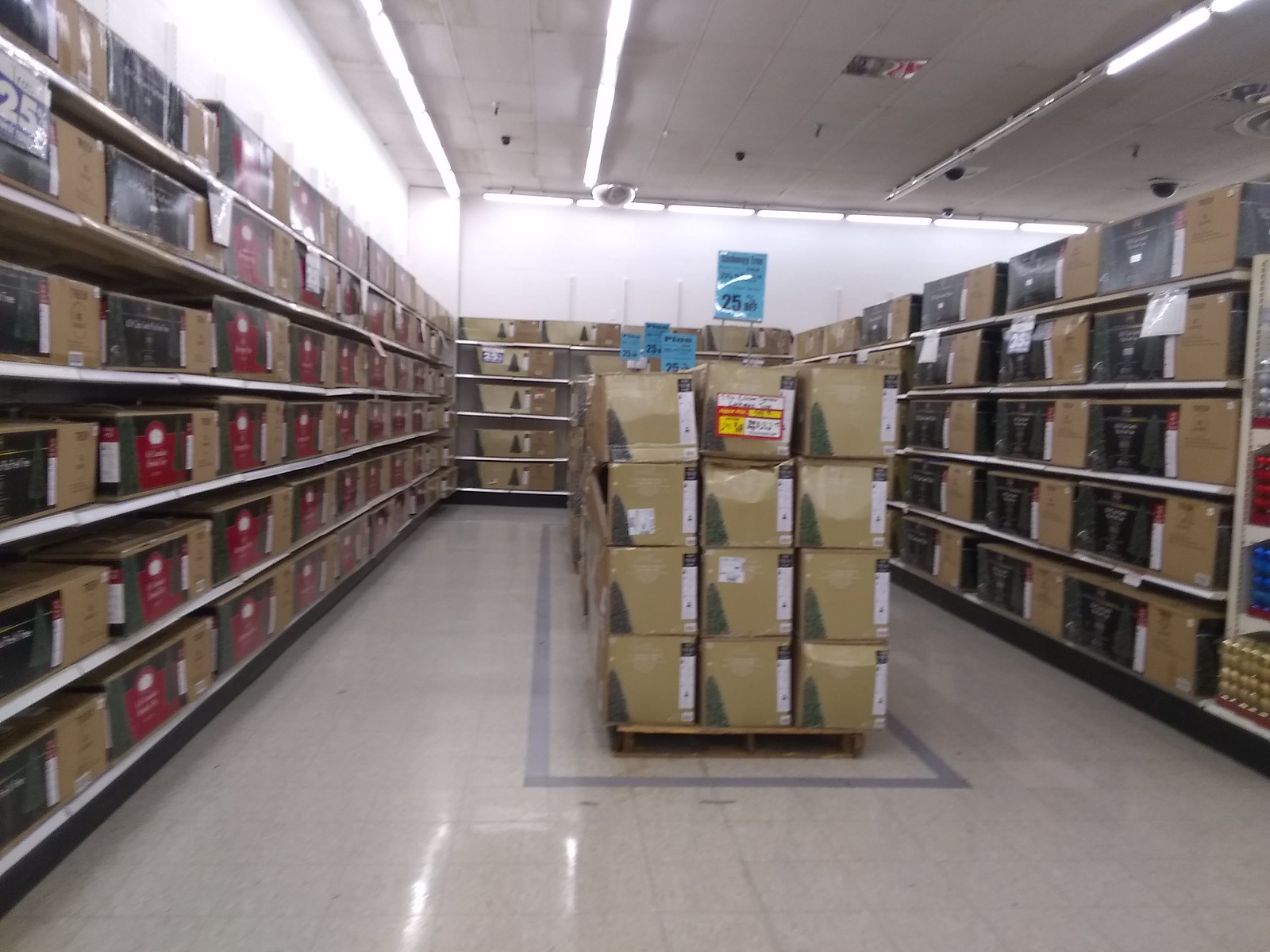This color photograph captures a scene in a retail store, reminiscent of an old Kmart, characterized by its plain white tile flooring and fluorescent lighting that creates a mix of highlights and shadows. The shelves lining the walls are a light beige metal and are stocked with cardboard boxes that appear to contain electronic equipment. Dominating the center of the image is a pallet, upon which a Christmas tree is spotlighted, suggesting that this section of the store is designated for holiday items. Overhead, banners hang from the ceiling, potentially advertising sales or promotions, adding to the bustling retail atmosphere.